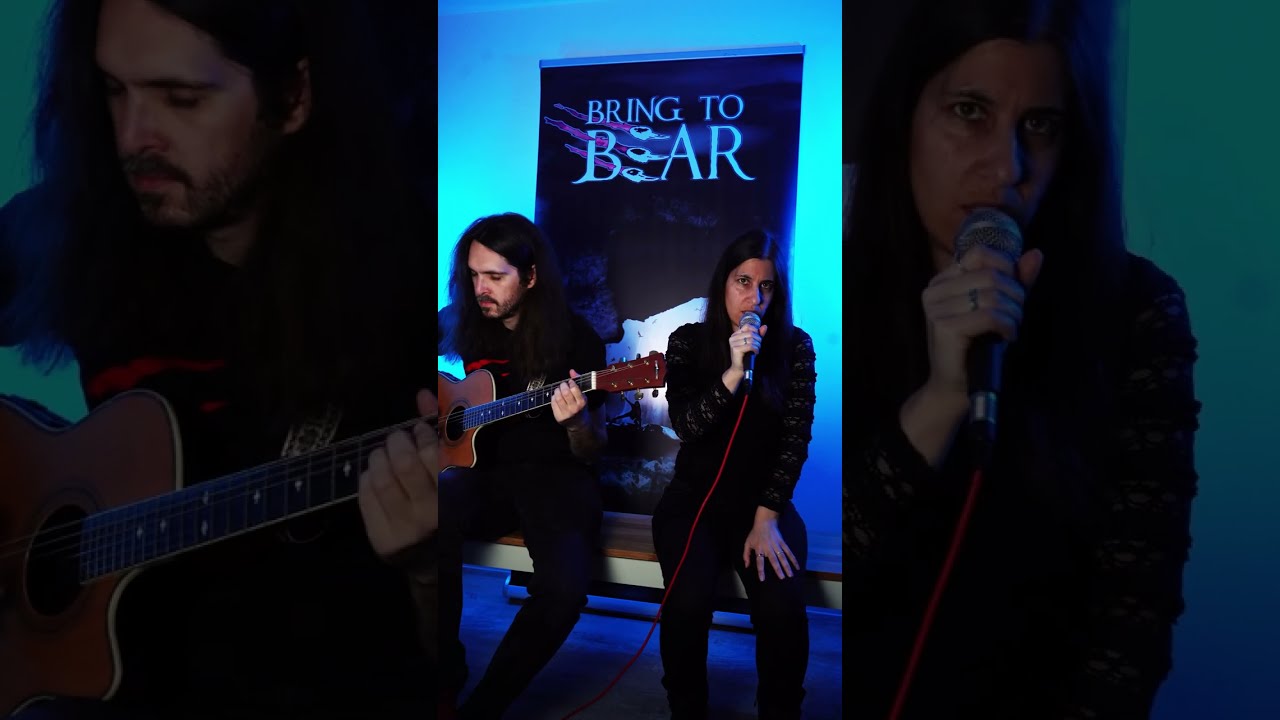In this photograph, two musicians are seated on a wooden bench with a white trim. The bench is positioned against a wall illuminated in blue light, which causes a soft, glowing effect on their sides. On the wall behind them, there is a poster that reads "Bring to Bear," with the 'E' in "Bear" stylized as a claw mark.

The musician on the left is a man with long, deep black hair, wearing an all-black outfit with mesh sleeves. He is playing an acoustic guitar with a brown body and a dark brown head. The musician on the right is a woman, also dressed entirely in black, holding a silver microphone with a red cable. Both are seemingly engrossed in their performance, suggesting an unplugged session or a small concert. The background fades into a blur, keeping the focus on the performers and the vibrant blue-lit wall behind them.